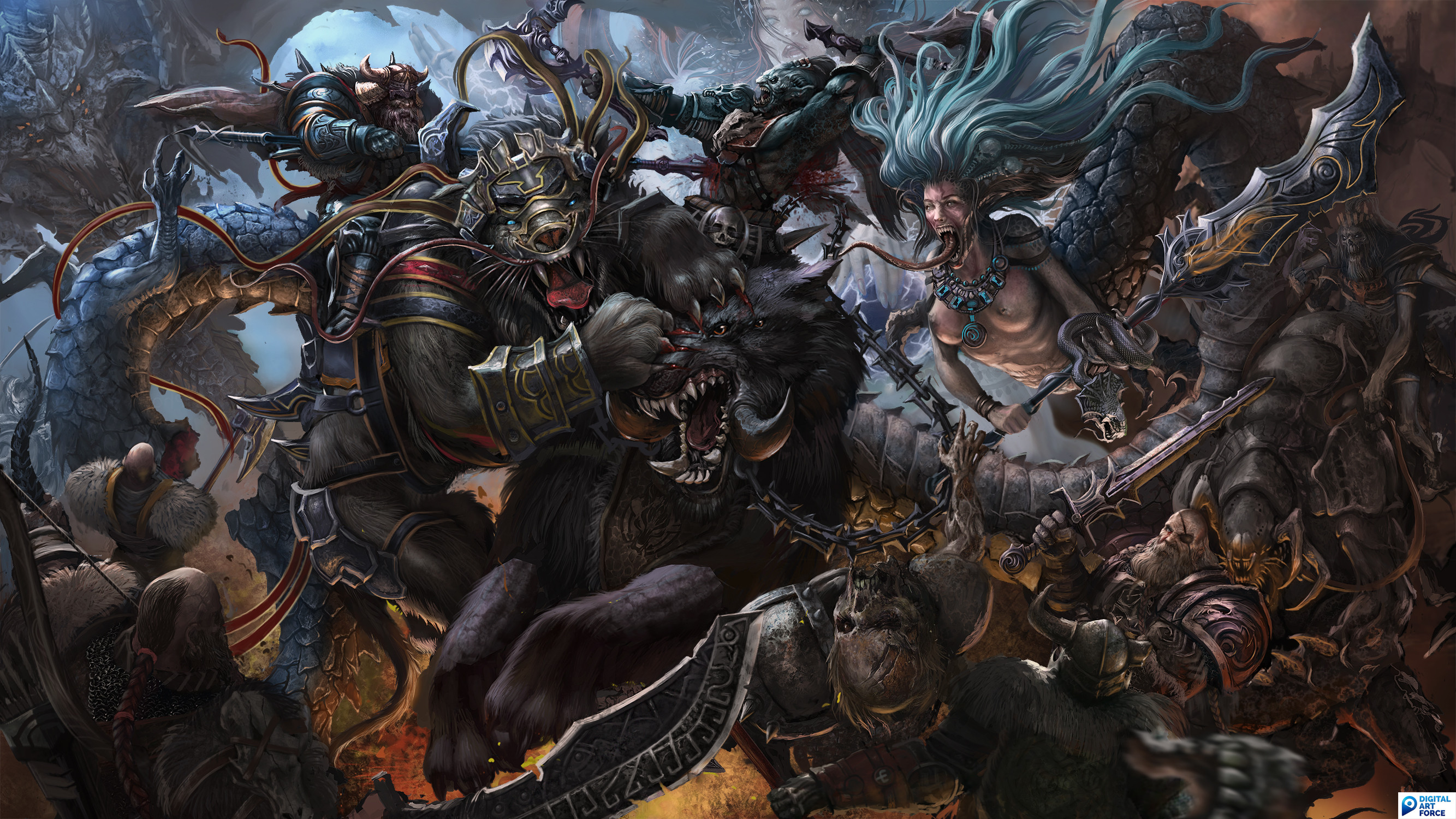In this highly detailed and dynamic image, we see what appears to be a scene captured mid-action, evoking the intensity of a slow-motion fight sequence often featured in movies. The artwork resembles a blend of comic book and cartoon styles, which could either be a traditional painting or an AI-created image. 

At the center of this dramatic scene, two beastly creatures are locked in a fierce battle. One beast is shown with its claws deeply embedded in the face of the other, showcasing the brutality of their confrontation. Adding to the surreal nature of the image, there is a striking figure of a woman who appears to be a blend of mythological entities—a Medusa and a mermaid. This hybrid character has blue-tinted skin and is notably not wearing a t-shirt, leaving her breasts exposed. She holds a knife, further intensifying the combative atmosphere of the scene. The overall composition captures the raw energy of a chaotic fight, freezing a moment of violent struggle in an artistically captivating manner.